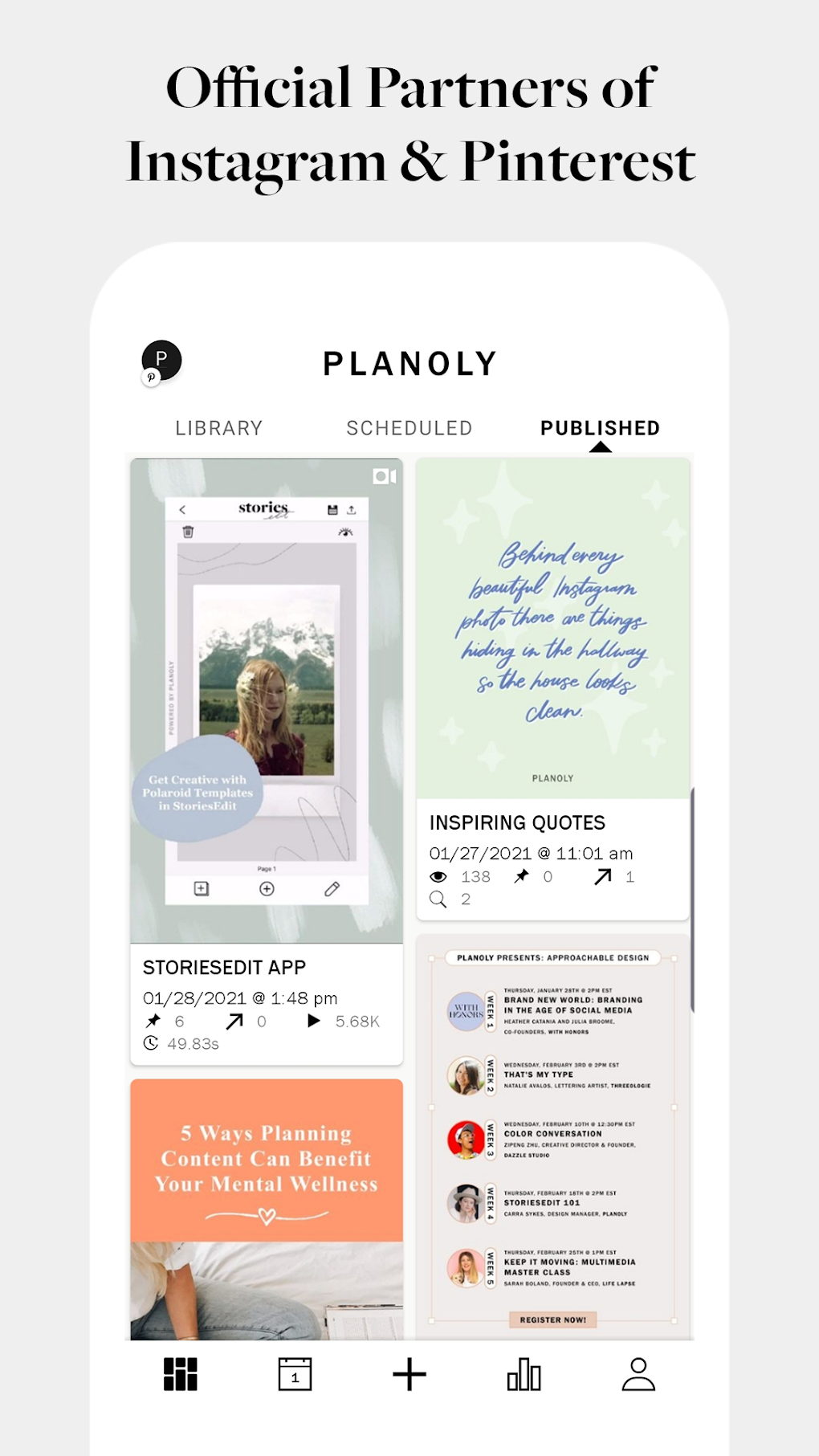In this image, we observe a detailed visual diagram highlighting a social media management tool. At the top, text denotes the tool as an official partner of Instagram and Pinterest. Below this heading, an outline of a smartphone is presented with the label "Plan Oli" prominently displayed at the top center of the phone screen. To the left, there is a black circle with a white letter "P" inside, accompanied by the Pinterest logo situated at the bottom left of the circle.

Further down, the interface is segmented into three tabs: Library, Scheduled, and Published, with the "Published" tab being the active selection. The screen displays a series of posts under this tab. The first post, positioned on the left, is titled "Stories Edit App" and was posted on January 28, 2021, at 1:48 PM. Following that, the next post is labeled "Inspiring Quotes," posted on January 27, 2021, at 11:01 AM. 

Two additional posts are partially visible at the bottom, their full details cut off by the screen's edge. One post features a picture on the left with text reading "Five Ways Planning Content Can Benefit Your Mental Wellness." On the right side, another post titled "Plangley Presents Approachable Design" includes various bullet points summarizing its content.